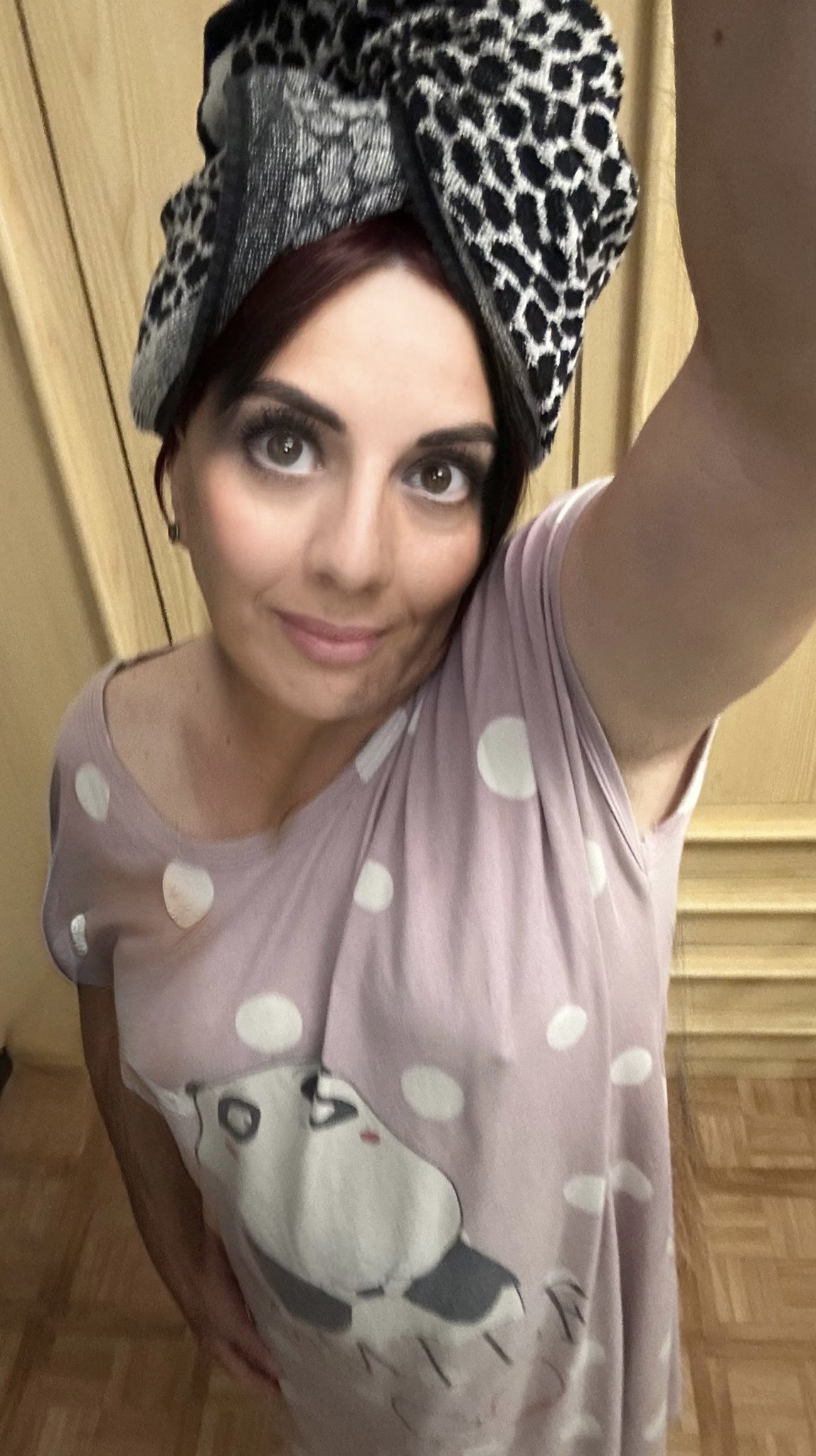In the image, a Caucasian woman in her late 30s or early 40s is taking a selfie using her phone. The photo has a tall, thin dimension, with the woman holding the phone above her head and looking up at the screen, resulting in no eye contact with the camera. She has light complexion skin, brown eyes, and brown hair that shows hints of auburn red, peeking out slightly from under a head wrap. The head wrap is prominently styled like a beehive and features a black and white leopard (or cheetah) print pattern.

Her makeup includes filled-in eyebrows, some white eye makeup on her waterline, and long, false eyelashes. She also wears pink lipstick and has a slight smirk with her lips closed. The woman is dressed in a loose, light purple pajama top adorned with large white polka dots and an illustrated panda bear, which might also include some text, though only the letters "L" and "F" are visible in black. 

In the background, you can observe a light wood floor with square patterns and darker brown lines around the edges. There is also a tall wooden cabinet or wardrobe behind her, adding to the cozy interior setting of the photograph.